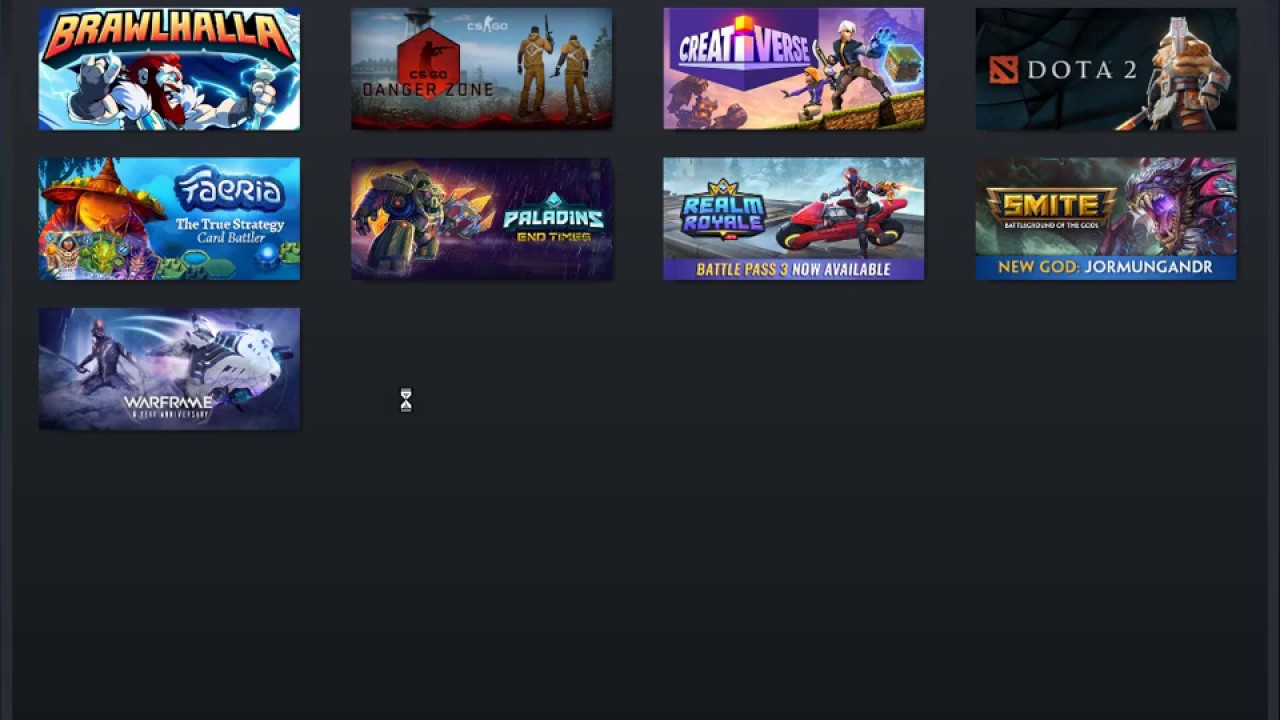The image features a black interface displaying an array of various video games, organized neatly into four rows. Each game is depicted with its respective artwork, title, and distinct colors representing different categories. From left to right, the games and details are as follows:

1. **Brawlhalla**: Prominently features white characters against a backdrop of blue, red, and white hues. The Brawlhalla logo transitions from yellow to red.

2. **Danger Zone**: The details of this game are not as vivid, but it follows next in the lineup.

3. **Creativerse**: Notable for its creative and exploratory elements, the specifics of its visual design are not detailed.

4. **Dota 2**: A highly popular multiplayer online battle arena game, known for its complex strategic gameplay.

5. **Tierra The True Strategy**: Depicts a strategic gameplay environment, although specific visual elements are not described.

6. **Carol Butler**: Details about this game are sparse in the description.

7. **Paladins**: Known for its team-based gameplay mechanics, similar to popular shooter games.

8. **End Times**: Specific visual details are not mentioned.

9. **Realm Royale**: Features a red motorcycle with a human rider clad in a helmet and motorcyclist outfit. It advertises the 'Battle Pass 3' as now available.

10. **Smite**: Showcases a new god character, Jormungandr.

11. **Warframe**: Presented as an active selection, indicated by an hourglass icon, suggesting the viewer is awaiting further options.

Each title's image serves as a preview, providing a glimpse into the diverse genres and gameplay experiences available within this collection.